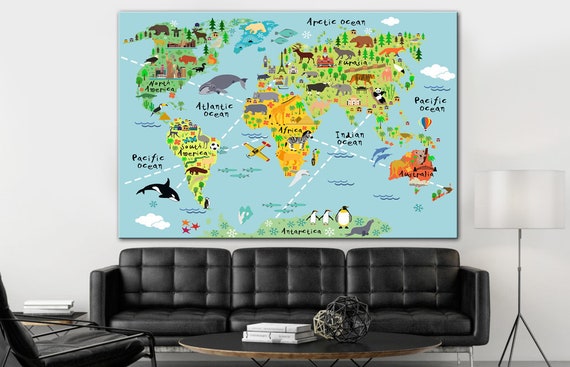The image depicts a modern living room featuring a centerpiece of a childlike, hand-painted canvas map of the world adorned with cartoonish illustrations of animals indigenous to each region. This vibrant and educational piece, characterized by blues, greens, and yellows, is mounted on an off-white wall above a large black leather sofa with three seating sections and quilted cushions. The sofa, with its more rigid sides, is accompanied by a sleek black-topped wooden coffee table, on which sit two spherical sculptures and a stack of white books. To the right of the sofa stands a floor lamp, distinguished by its white lampshade and black tripod base. On the left side of the room, a matching black leather chair completes the seating arrangement, encapsulating a cozy and educational atmosphere reminiscent of a child's room.